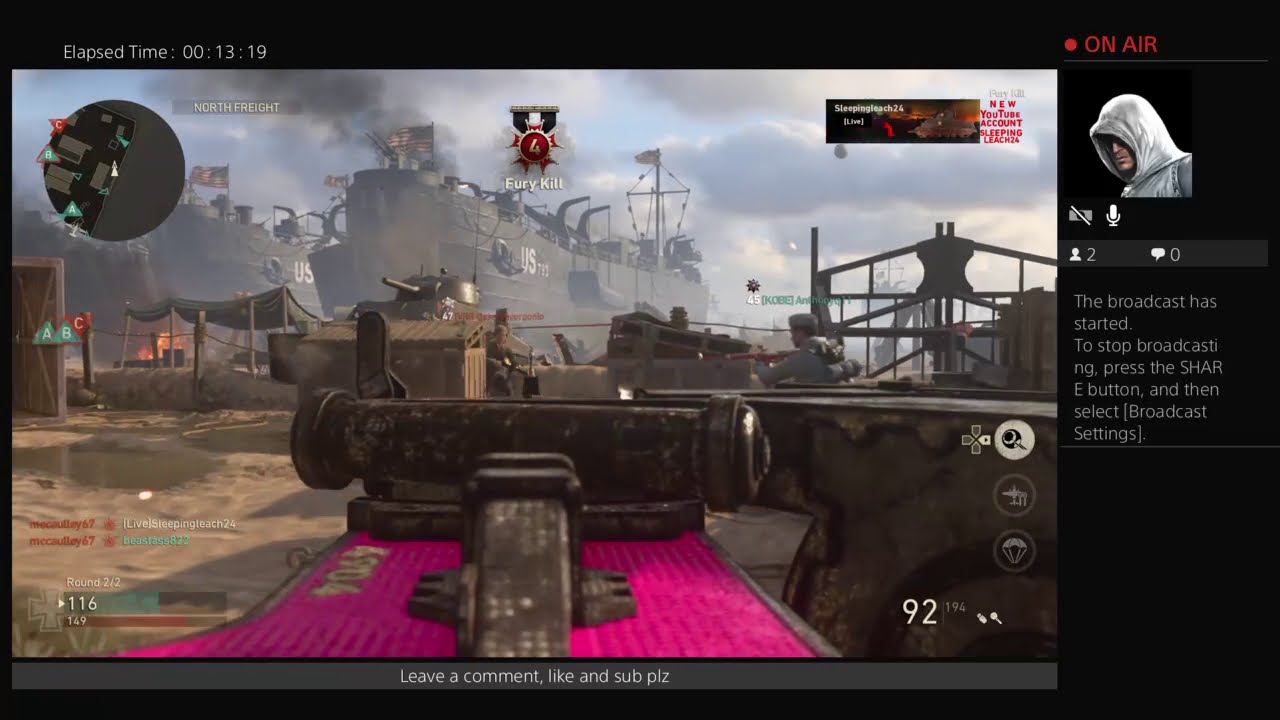The screenshot presents an in-game scene from a live-streamed war-themed video game. Dominating the image is a dramatic battlefield under a hazy sky with white fluffy clouds and billowing smoke. In the foreground, a weapon points towards massive, old-style warships, evocative of historical American naval vessels, engaged in combat. These ships, along with other wooden and metal military vehicles, create a chaotic war zone on a landscape featuring a bright pink and red brick road flanked by dirt terrains and a brown tent on a hill. There's a small fire behind the tent. 

On the right side of the screen, a black strip displays a photo of a man in a gray hooded sweatshirt, presumably the live-stream commentator, partially obscured. Below his image, various game stats and white text about the broadcast appear, including a directive to leave a comment, like, and subscribe. The upper left corner showcases a game timer and an animated character within a black circle. The bottom section of the screen reiterates the call to action: "Leave a comment, like, and sub, please." This vivid, color-rich screenshot exemplifies a typical freeze frame from the ongoing adventure and strategic gameplay being aired live.